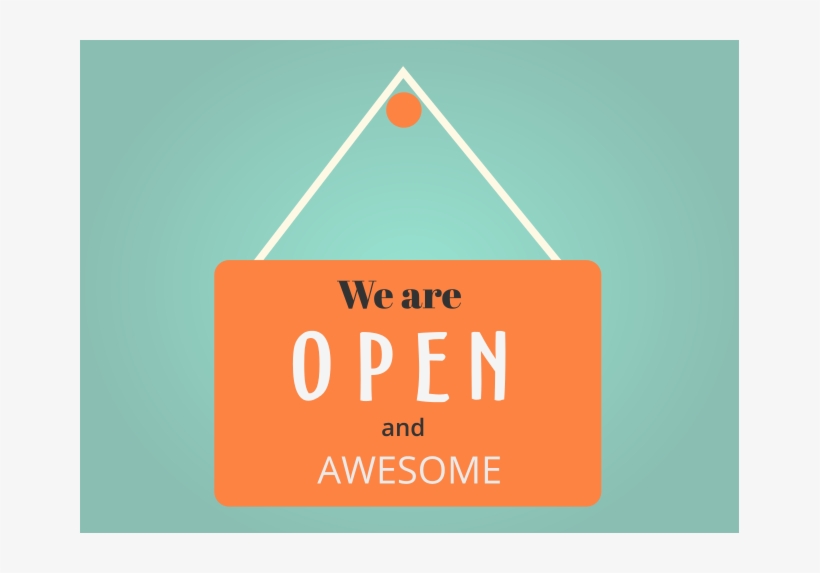The image features an illustration of a store sign set against a light blue-green backdrop, framed within a light gray border. The sign is centrally positioned on the background and is depicted as being hung by a white string from an orange pin or nail, which creates an angular, triangular shape rather than a curved string. The sign itself is an orange rounded rectangle with a series of texts in black and white font. At the top, in black ink, it reads, "we are," followed by the word "open" in bold, larger white text. Beneath that, in smaller black text, it says "and," and finally, in a different font and white text, it proclaims "awesome." The overall aesthetic emphasizes a welcoming and vibrant message with a clear and bold design.